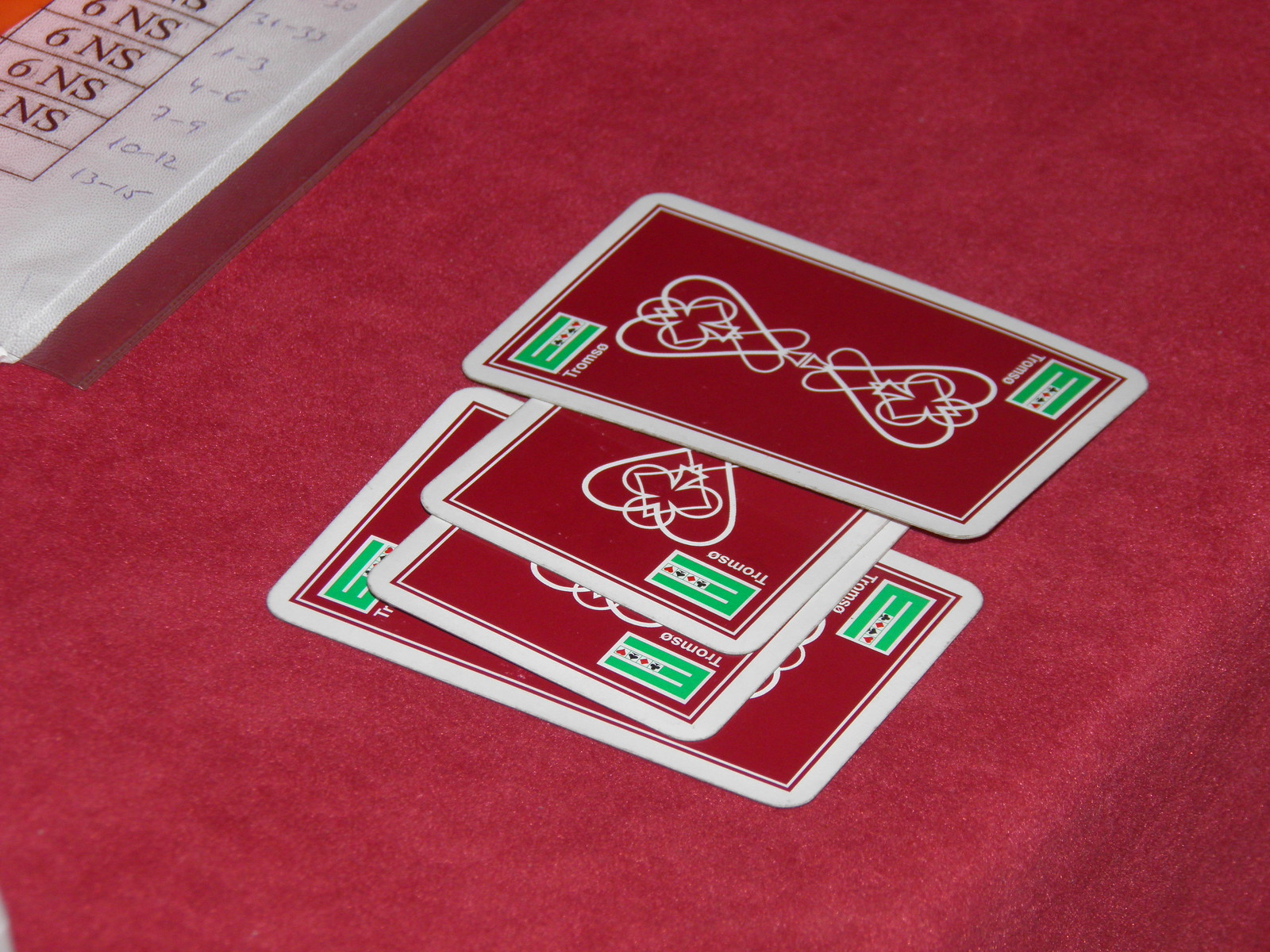On a table draped with a vibrant red felt tablecloth, a neatly arranged stack of playing cards takes center stage. The tablecloth is securely fastened to the table, ensuring it remains smooth and unwrinkled. The stack consists of four cards, methodically placed one on top of the other. Each card features a pristine white border, framing the rich red center. Intricately designed heart-shaped figures, reminiscent of a complex fusion of hearts, clubs, and diamonds, adorn the middle of the cards, creating an elaborate pattern. Green sections are present at the top and bottom corners of each card, accentuated with touches of white, adding to the intricate design.

Above the cards, positioned at the top of the photograph, lies a piece of paper, likely a scorecard. The paper lists numbers 2-9, 10-12, and 13-15, hinting at the progression of a card game. The cards themselves are face down, obscuring their identities and adding an element of mystery to the scene. The overall setup suggests an ongoing or recently concluded card game, captured with meticulous detail in this photograph.